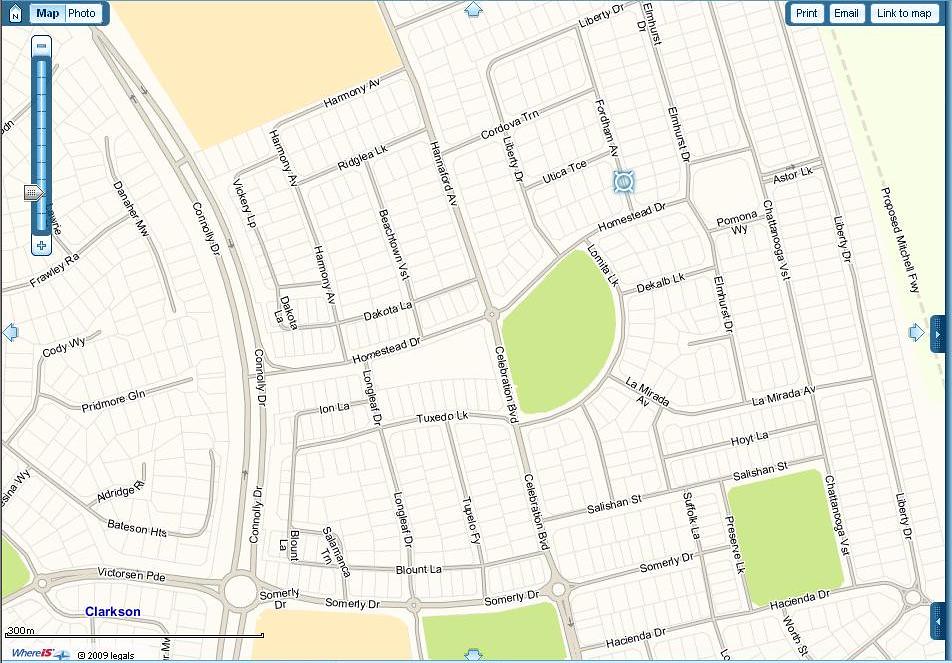This graphic GPS map provides a detailed view of an unidentified location, with no time or date specified for the search. The map is depicted in a graphic format rather than a satellite view. Various areas are color-coded, with green indicating parks and recreational spaces, while most other areas are highlighted in light yellow with road markings overlaid. Key roads in the central part of the map include Hartford Avenue, La Miranda Avenue, DeKalb Lane (appearing twice), Boudicca Toe, Homestead Drive, Dakota Lane, Beachtown, and Longleaf Drive. Additionally, there is a proposed Michael Freeway marked on the map. Above the map scale, the name "Clarkson" is displayed, possibly indicating the name of the area or city. However, there is no pin or marker identifying the specific city.